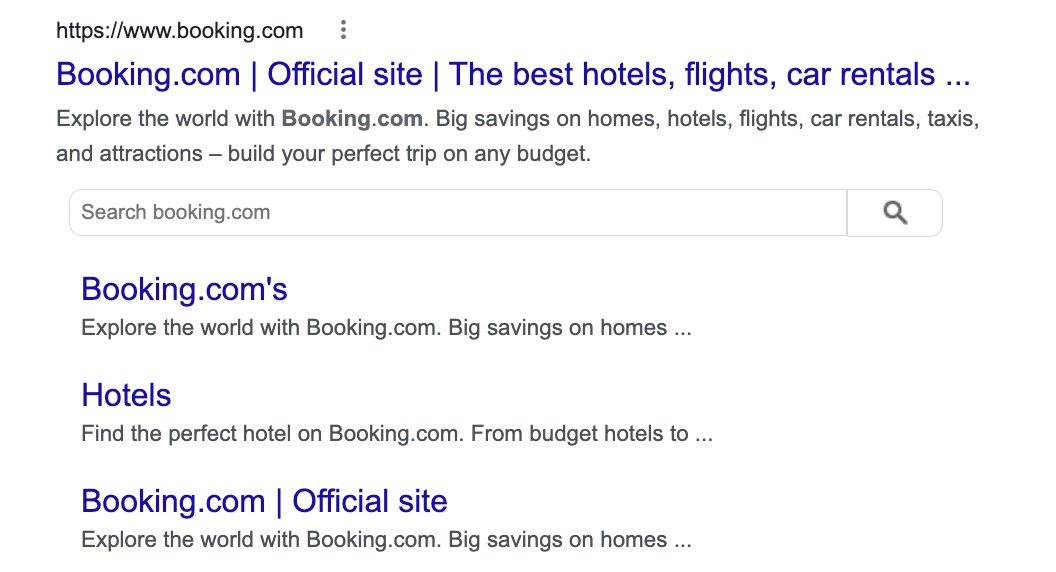This detailed snippet from a search result page for Booking.com provides a comprehensive overview of the site's offerings and functionalities. 

In the upper left corner, the black text "HTPS Booking.com" is displayed, accompanied by three vertically aligned dots to its right. Directly beneath this, a blue headline reads "Booking.com | Official Site | The Best Hotels, Flights, Car Rentals..." This is followed by a bolded black description that encapsulates the site's services: "Explore the world with Booking.com. Big savings on homes, flights, hotels, car rentals, taxis, and attractions. Build your perfect trip on any budget."

Below this descriptor, there is a search bar centrally labeled with gray text instructing users to "Search Booking.com." This search bar includes a magnifying glass icon and a vertical dividing line towards its right side.

Additionally, three sub-results are outlined beneath the primary search result. Each sub-result begins with a blue header. The first is titled "Booking.com's hotels," followed by gray subtext: "Explore the world with Booking.com, big savings on homes..." The second header, "Booking.com | Official Site," is accompanied by black subtext: "Find the perfect hotel on Booking.com from budget hotels to..." The third header mimics the first, repeating: "Explore the world with Booking.com, big savings on homes..."

This snippet provides a clear, detailed representation of what users can expect when navigating the Booking.com site, emphasizing its wide range of travel-related services and user-friendly search functionality.